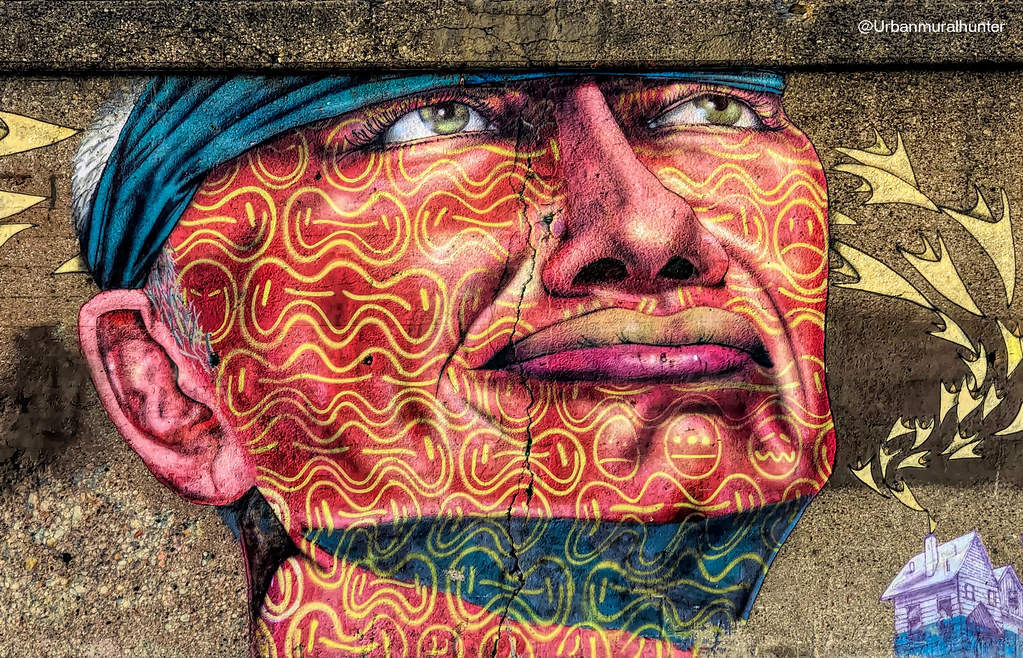This detailed image captures a striking piece of street art, likely a mural found in an urban setting, as suggested by the small white lettering in the upper right corner that reads "Urban Mural Hunter." The artwork, painted on a cracked concrete surface with a dark, dirty creamish-tan texture, portrays the close-up of an older man's face, his features marked by subtle wrinkles. He gazes slightly upward and to the right, a thoughtful expression on his face.

The man's skin is depicted in an abstract, layered pattern of reds and yellows, with additional texture provided by squiggly pink lines resembling stretched-out happy faces. His facial shadows are rendered in blues with a similar yellow squiggly texture design, and parts of his neck in greens and blues. His pink ears and lips, alongside a purplish nose, add further depth to his visage. Short white hair peeks out from beneath a blue bandana wrapped around his forehead.

In the lower right corner of the mural, a small purple house with yellow triangular shapes representing smoke emanates from its chimney, adding an element of whimsy to the piece. The intricate details and mix of colors bring this street art to life, making it a captivating visual study.